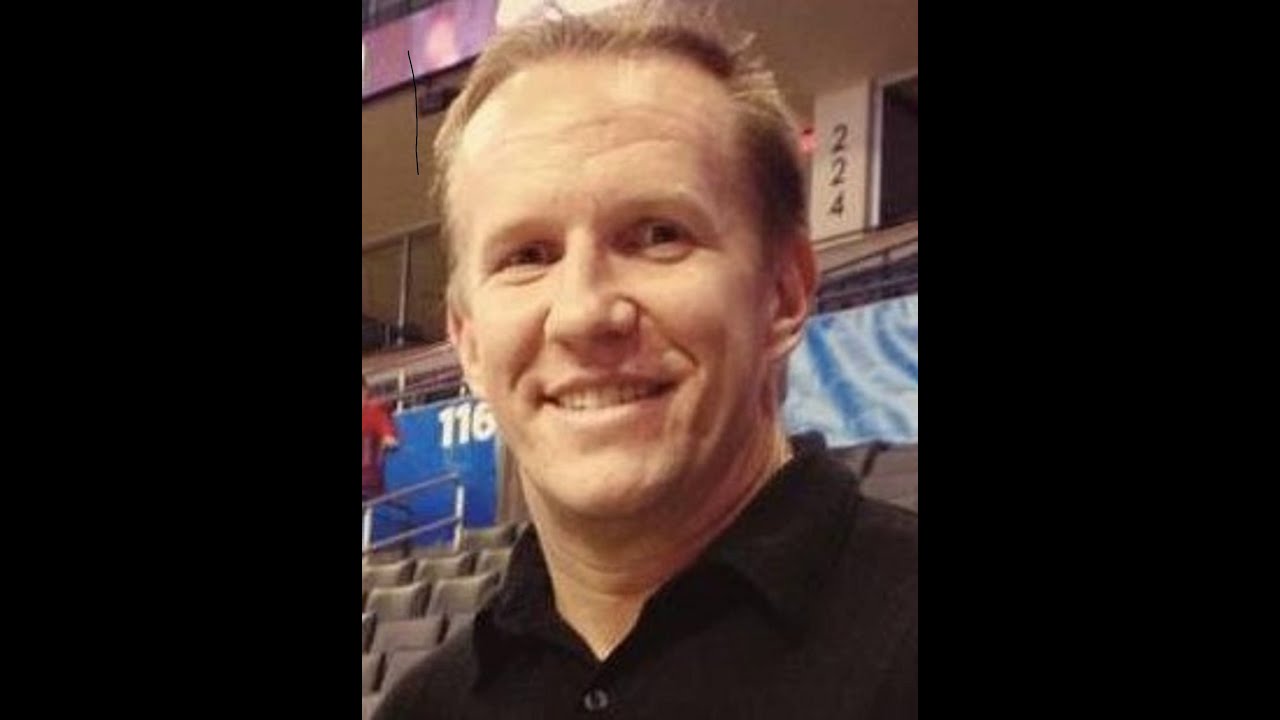The image prominently features a close-up of an older white man smiling directly at the camera. He appears to be in his fifties or early sixties, with short, thinning, light brown hair and some wrinkles, particularly noticeable on his neck. He's dressed in a black button-up shirt and his smile reveals a straight white top row of teeth. The background suggests he is at a sporting event, as he is seated in what looks like a stadium or bleachers, with black seats ascending behind him. Above and around him, various signs and numbers are visible, including "116" to the left of his head and "224" on a pillar above him. Additional elements in the background include advertisements on LED screens, guardrails, and possibly an exit sign, all contributing to the stadium-like atmosphere. The image is filled with colors like blue, black, white, and hints of other shades in the surroundings, reinforcing the setting of a large public venue.